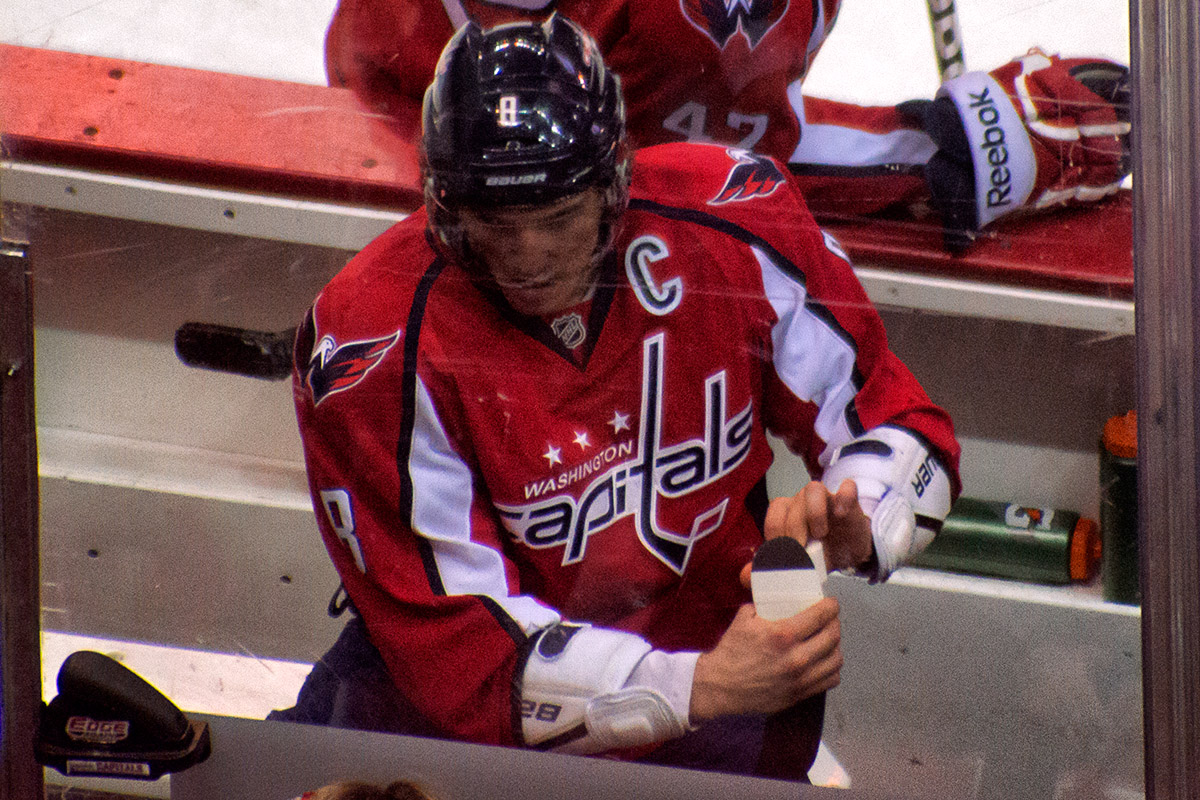The image captures a detailed moment during a Washington Capitals hockey game. The focal point is the team's captain, marked by the "C" on his predominantly red jersey with white and black accents. His attention is drawn downward, possibly towards his hockey stick, suggesting he might be adjusting or checking it. The captain's jersey features the team's name, "Washington Capitals," in dark lettering with three white stars above "Washington," and his number, 8, is visible on his sleeve. He is wearing black or dark blue pants, white cuffs, and a black helmet. In the background, another Capitals player is seated, while a third player, partially visible, stands on the ice with a large glove and the number 42 or 47 on his sleeve. The setting includes typical rink surroundings, with concrete flooring and a few green and orange Gatorade bottles nearby. The overall ambiance indicates this scene is from an ongoing game rather than a practice session.